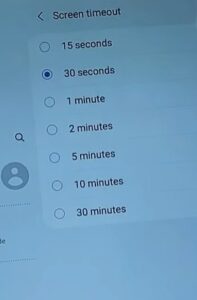The image is a screen capture of a portion of a computer desktop screen, slightly tilted diagonally. The background is blue, while the text is black. At the top of the image, the heading "Screen Timeout" is prominently displayed. Below this heading, a list of options specifies various time intervals for screen timeout settings. These options are arranged in ascending order of duration: 15 seconds, 30 seconds, 1 minute, 2 minutes, 5 minutes, 10 minutes, and 30 minutes. The option for "30 seconds" is selected, indicated by a checked radio button positioned to the left of the "30 seconds" option.